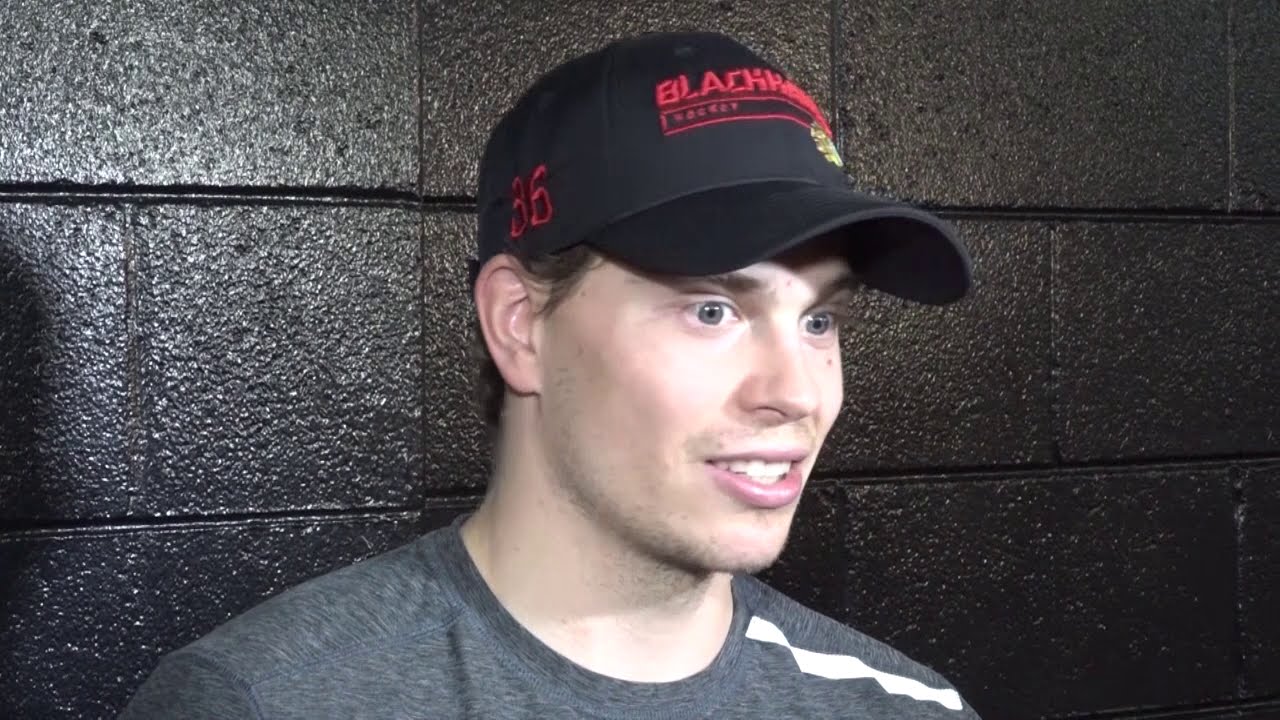The image captures a young, white-skinned gentleman in what seems to be a candid moment, possibly during an interview. He is glancing to the right, revealing a profile of his face. He sports a black baseball cap, prominently featuring the word "Blackhawks" embroidered in red on the front and the number "36" on the left side. His cap partially obscures his dark brown hair. The man's eyes appear brown, with some descriptions suggesting a grayish tint. His facial hair includes a budding mustache and a bit of growth on his chin. His mouth is slightly open, exposing both his upper and lower teeth, suggesting he might be in mid-conversation or smiling. He is dressed in a gray t-shirt accented with a distinctive white stripe along the left shoulder. The setting is against a backdrop of dark, concrete block walls, painted black, adding a stark contrast to his attire and making the red details on his cap more striking.